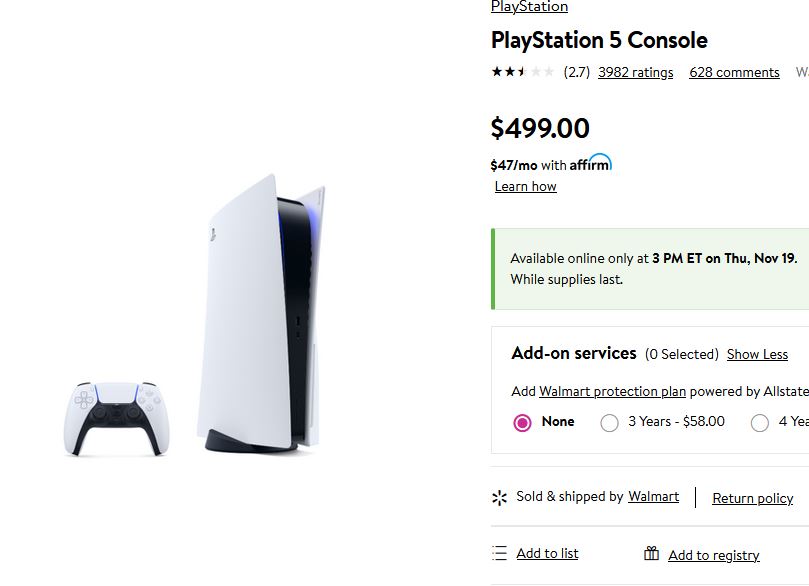The screenshot from Walmart.com features the sale page for a PlayStation 5 console. On the left side, there is a high-resolution image of the console, showcasing its sleek white design with a matching white controller. The console stands vertically on a black stand, resembling a white sandwich cookie with a black center, adorned with blue LED lights.

On the right side, detailed information about the product is presented. The title "PlayStation 5 Console" is prominently displayed, followed by a rating of 2.7 out of 5 stars based on 3,982 ratings and 628 comments. The price is listed as $499, with an additional financing option of $4.87 per month through Affirm, highlighted by an underlined "Learn how" link.

Below the price information, there is a gray box with black text stating the availability details: "Available online only at 3 p.m. Eastern on Thursday, November 19th, while supplies last." A brief commentary suggests the low rating is justified.

The page also notes that no add-on services are available and the product is sold and shipped by Walmart.